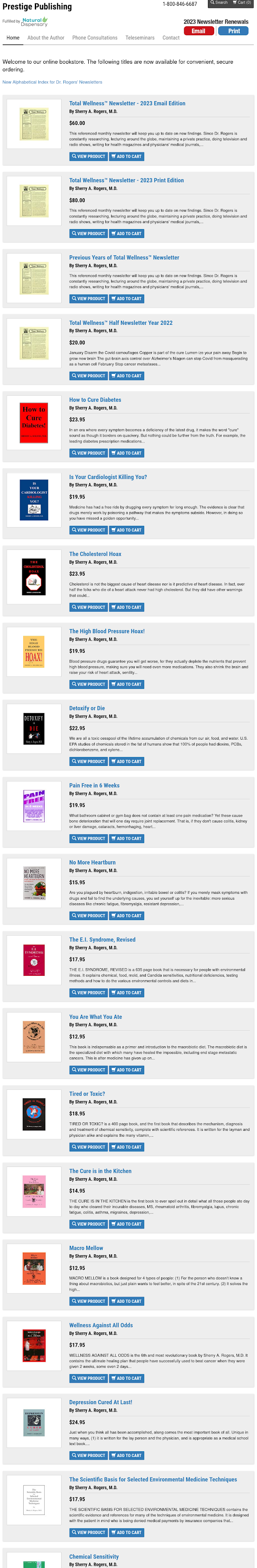The image features a structured layout with a total of 19 horizontal rows, each separated by a gray bar. In the upper left-hand corner, "Prestige Publishing" is prominently displayed in boldface type. On the left side of each row, there is an image enclosed in a white box, while the right side contains a blue title. Below each title, there appears to be a description, although the text is quite small and challenging to read. Each row also includes two buttons aligned to the left. At the very top of the image, there are multiple buttons, including a red button and a blue button located in the upper right-hand corner. Additionally, there's a black box with indeterminate content, and to its left, a phone number is displayed. The design maintains uniformity, with all item boxes being of identical size, giving the overall layout a very regular and orderly appearance.